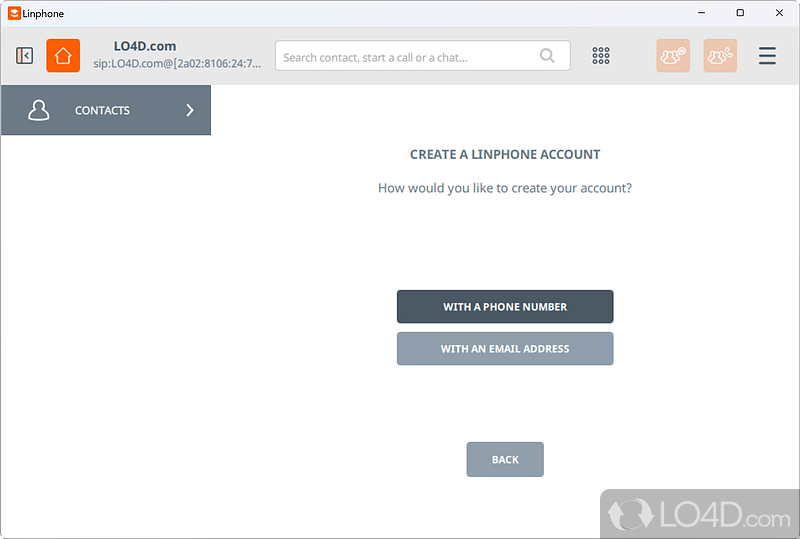The image is a screenshot of a webpage displayed on a computer. 

**Top Section:**
- At the very top, there's a light-colored bar. 
- On the left-hand side of this bar, there's an orange square with a white logo to its right, accompanied by the black text "Linphone."

**Below the Top Section:**
- Just beneath the light-colored bar, there's a darker gray bar.
- On the left side of this darker gray bar is another orange square with a white house outline. Next to this icon, it reads "LO4D.com, SIP: LO4D.com @ (2A02:8106:24::7...)" in black font.
- A white search bar is situated in the middle of this darker gray bar, flanked by some icons.

**Left Sidebar:**
- The left quarter of the screen features a vertical gray bar.
- At the top of this bar is an outline of a person icon, along with the word "Contacts" in white text and a white arrow pointing to the right.

**Central Section:**
- In the center of the screen, large text reads "Create a Linphone account. How would you like to create your account?"
- Below this prompt, there are two options:
  - A black bar that says "With a phone number" in white text.
  - A gray bar that says "With an email address," also in white text.
- Further down, there is a small gray button labeled "BACK" in large white letters.

**Bottom Section:**
- In the bottom right corner of the screen, there is a logo adjacent to a light-colored or gray bar. This bar contains the text "LO4D.com."